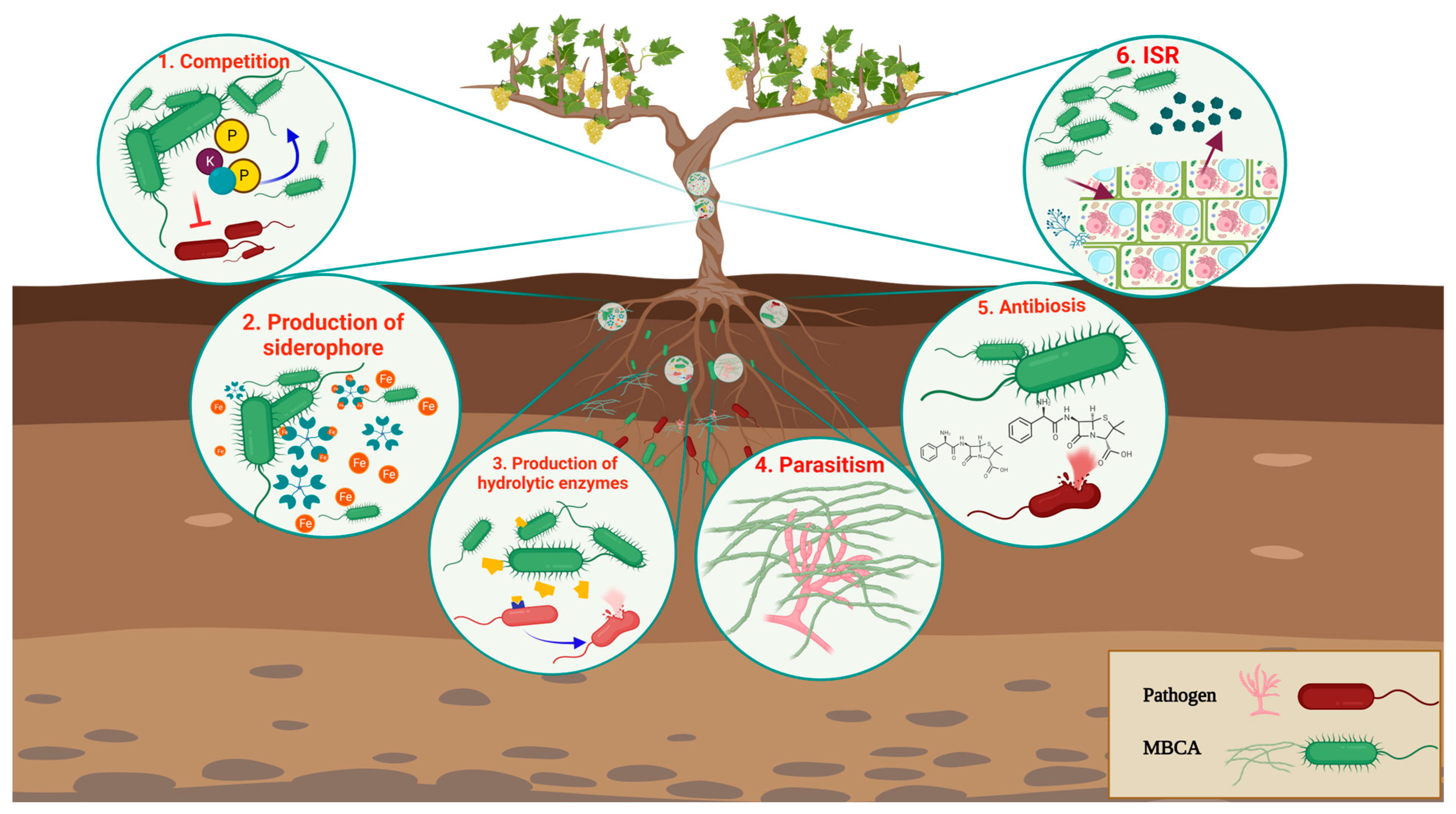This detailed scientific illustration depicts a tree with its roots extending deeply into the ground, interspersed with various strata of soil that transition from dark to increasingly lighter shades, punctuated by layers containing stones. The tree, complete with two branches adorned with green leaves and some yellow fruit, serves as the focal point. Surrounding the tree are six intricately labeled circular diagrams, each connected via lines to different parts of the tree, including both the trunk and the roots, highlighting various biological interactions and processes.

1. **Competition**: Depicted with several green oblong shapes and small circles indicating movement, this diagram illustrates the competitive interactions among microorganisms with red-letter labeling.
2. **Production of Siderophore**: This section visualizes a chemical process, highlighting the role of siderophores in microbial activity.
3. **Production of Hydrolytic Enzymes**: Shown with multicolored representations of germs, this diagram indicates the enzymatic activity taking place.
4. **Parasitism**: Illustrated with images resembling green and red seaweed-like structures, this circle depicts the parasitic relationships within the soil ecosystem.
5. **Antibiosis**: Featuring green and red bug-like germs, this diagram visualizes the antagonistic interactions between microorganisms.
6. **ISR (Induced Systemic Resistance)**: This section shows green germs and blocks with arrows, representing the process of induced systemic resistance.

In the lower right corner, a key distinguishes the various elements: red shapes denote pathogens, while green shapes represent MBCA (unspecified in detail), including green seaweed-like figures and tablet-shaped germs. This color-coded legend aids in interpreting the microorganism interactions and their significance in the tree's ecosystem. Together, these elements offer a comprehensive view of the complex biological and chemical processes that influence the health and growth of the tree.